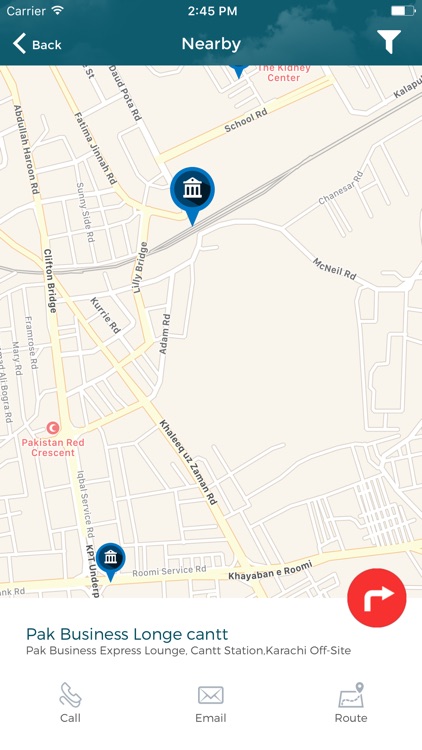A detailed image caption based on the given description could be:

"This phone screen capture prominently features a map. At the top of the screen, a teal bar contains navigation options: 'Back' on the left, 'Nearby' in the middle, and a cone-shaped icon on the right. The map itself is primarily beige, denoting the land, with roads highlighted in a yellowish-orange color. Significant landmarks include 'Curry Road,' 'Pakistan Red Crescent,' 'Seaman Road,' and 'Cambodian Rumi.' Towards the bottom of the screen, various locations are labeled: 'Pack Business Lounge,' 'Can't Station,' 'Karachi Offsite,' and 'Pack Business Express Lounge.' Users have quick access options for 'Call,' 'Email,' and 'Route,' each represented by their respective icons. Additionally, a white turn arrow within a red circle is visible, possibly indicating a navigation or direction feature."